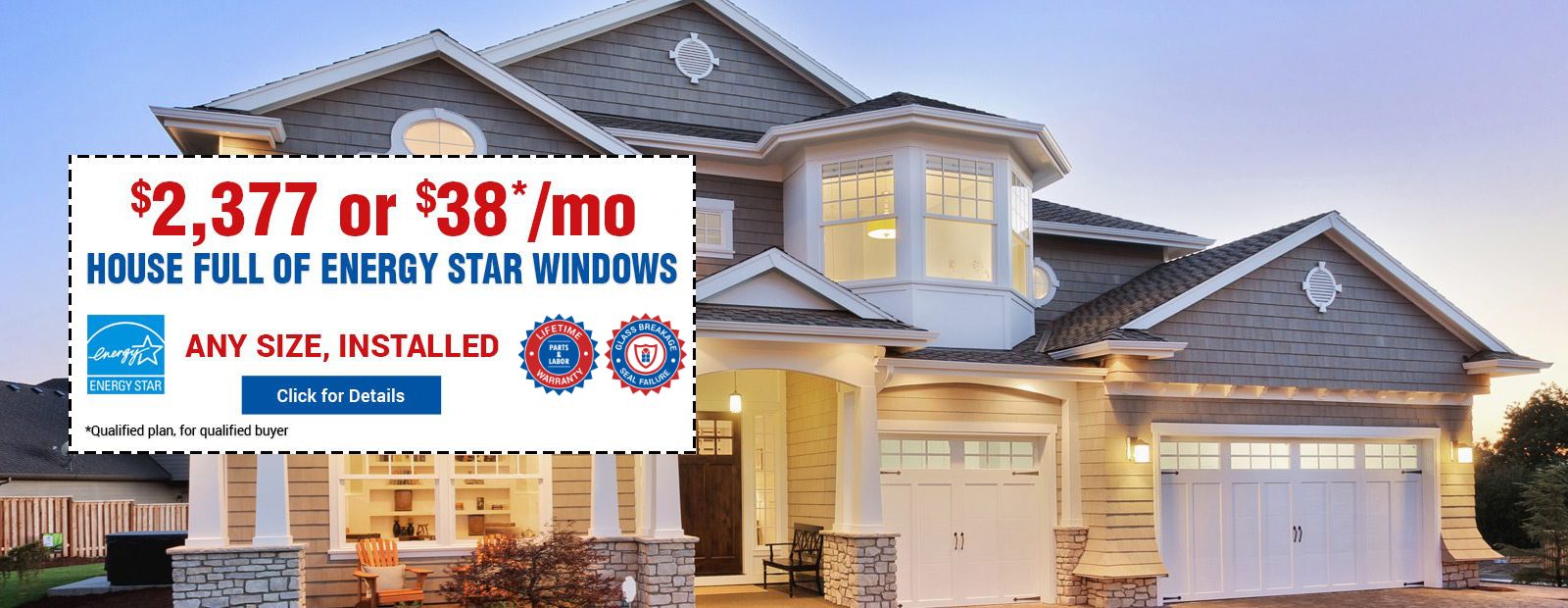The image depicts a close-up, rectangular photo of a two-story house set against a bright blue sky. The house features a gray and white exterior, with a bit of a front porch supported by elegant pillars. On the right side, there are two garage doors: a double garage door furthest from the house and a single one closest to it. To the right of the house, a bush is visible.

On the left side of the image, a centrally placed white rectangle, outlined with a black dashed line, contains important information. At the top of this rectangle, the text "$2,377 or $38* / MO" appears in large, bold red font. Below this, in dark blue all-caps, is the phrase "HOUSE FULL OF ENERGY STAR WINDOWS." Two lines beneath, on the left side, there is a blue square with the Energy Star logo. Centered and to the right, in red all-caps, the text reads "ANY SIZE, INSTALLED." Adjacent to this, two seals are visible. At the bottom of the rectangle, a blue rectangular button says "CLICK FOR DETAILS" in white font.